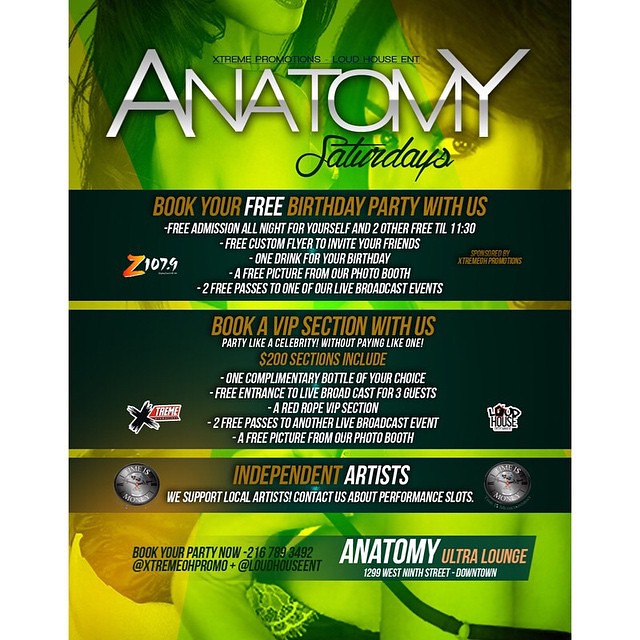The advertisement is a vertically-oriented, computer-generated design dominated by shades of green and brown. At the top, the image subtly features the eyes and part of the hair of two women, creating a mysterious and sophisticated aura. The prominent text at the top reads "Anatomy Saturdays" in bold lettering, and emphasizes the availability of free birthday party bookings.

Below, a black bar hosts crucial details in white and brown text: "Book your free birthday party with us. Free admission all night for yourself and two others. Free until 11:30." Additional information highlights a VIP section for $200, which includes various perks like one complimentary bottle of choice, free entrance to live broadcast events for three guests, a red rope VIP section, two free passes to another live broadcast, and a picture from the photo booth.

Prominently featured are details about supporting local independent artists, encouraging contact for performance slots. The venue is identified as "Anatomy Ultra Lounge" located at 1299 West 9th Street downtown, with sponsorship by Z107.9. The incentive to party without paying high prices and enjoy music from independent artists is strongly emphasized, making it clear this is a vibrant and inclusive nightlife spot, reminiscent of a trendy club atmosphere.